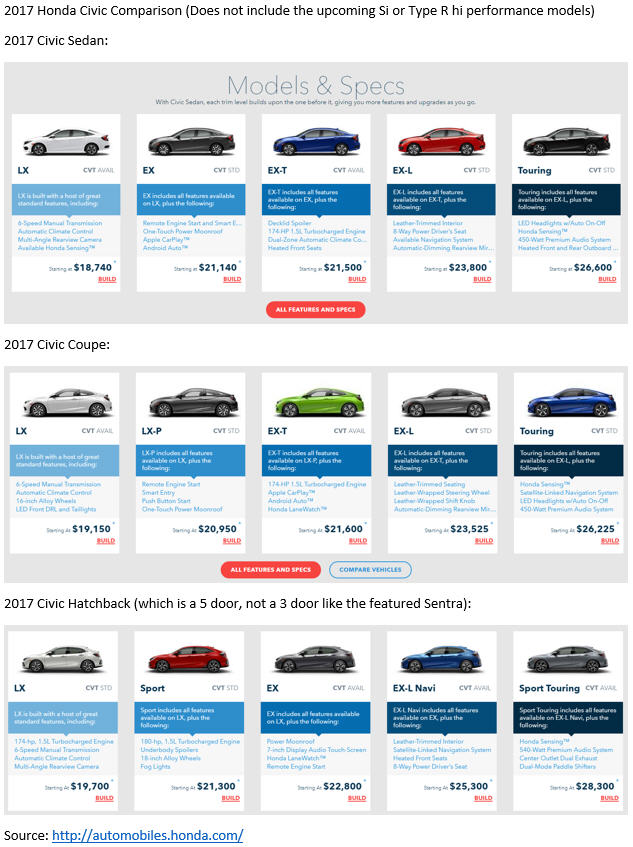Screenshot of a "2017 Honda Civic Comparison" Chart from automobiles.honda.com

The image is a screenshot from the website automobiles.honda.com, depicting a detailed comparison chart titled "2017 Honda Civic Comparison." Note that the upcoming SI and Type RHI performance models are not included in this comparison. The chart is organized into three distinct rows, featuring the 2017 Honda Civic Sedan, Coupe, and Hatchback models, respectively.

**2017 Honda Civic Sedan:**
1. **LX**:
   - Color: White
   - Starting Price: $18,740
2. **EX**:
   - Color: Black
   - Starting Price: $21,140
3. **EX-T**:
   - Starting Price: $21,500
4. **EX-L**:
   - Color: Red
   - Starting Price: $23,800
5. **Touring**:
   - Color: Black
   - Starting Price: $26,600

**2017 Honda Civic Coupe:**
1. **LX**:
   - Starting Price: $19,150
2. **LX-P**:
   - Color: Black
   - Starting Price: $20,950
3. **EX-T**:
   - Color: Green
   - Starting Price: $21,600
4. **EX-L**:
   - Starting Price: $23,525
5. **Touring**:
   - Color: Blue
   - Starting Price: $26,225

**2017 Honda Civic Hatchback:**
1. **LX**:
   - Starting Price: $19,700
2. **Sport**:
   - Starting Price: $21,300
3. **EX**:
   - Starting Price: $22,800
4. **EX-L Navi**:
   - Starting Price: $25,300
5. **Sport Touring**:
   - Starting Price: $28,300

Each price point features a link labeled "build" for potential buyers to start their customization process. Additionally, there are buttons beneath each car model for "all features and specs" and, in the case of the Coupe and Hatchback rows, an extra button for comparing vehicles. Note that the text descriptions accompanying each vehicle in the chart are slightly blurry and challenging to read. The 2017 Honda Civic Hatchback is specifically noted as a five-door model, contrasting the featured Sentra, which is a three-door vehicle.